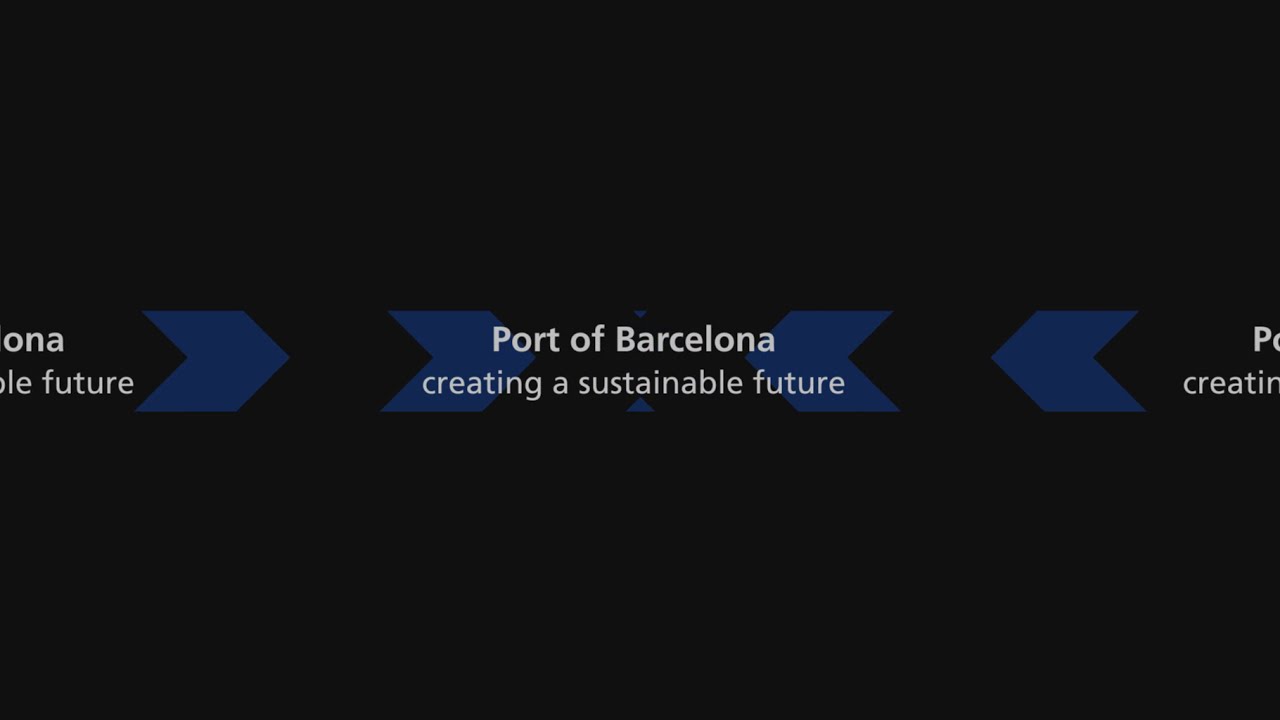The image is a black rectangular advertisement for the Port of Barcelona, emphasizing a sustainable future. Dominating the visual are four thick, dark blue arrows: two on the left pointing right and two on the right pointing left, converging towards the center. Across these arrows, in crisp white lettering, is the message: "Port of Barcelona, creating a sustainable future." Some of the text is partially cropped at the edges, reiterating the slogan on both sides. The stark contrast between the black background and the blue arrows, combined with the repeating white text, creates a bold and focused visual statement.